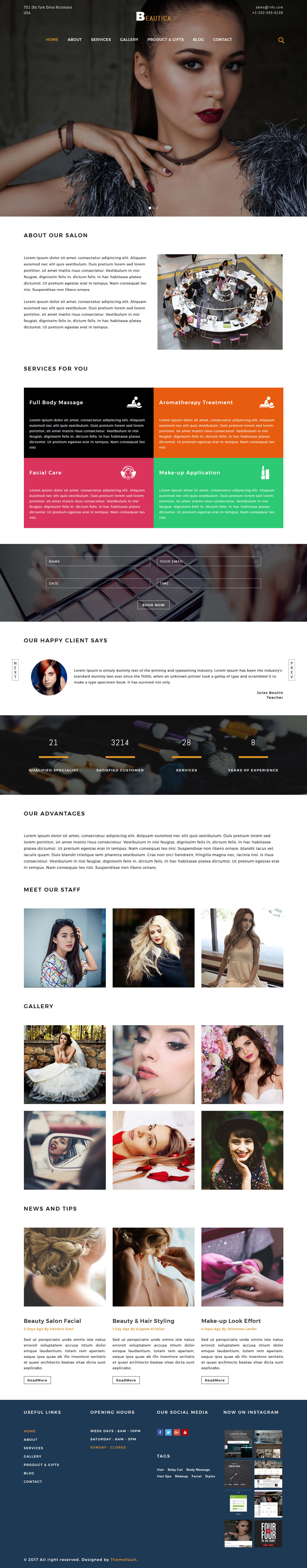This is a detailed description for a website showcasing salon services called "Utica." At the top of the website, there is a navigation bar with links to Home, About, Services, Gallery, Products and Gifts, Blog, and Contact. The main banner features a stunning woman with a natural makeup look complemented by striking red lipstick. She is wearing a stylish bracelet, and her nails are impeccably done in a chic white and red design.

Below this banner, there is an "About Our Salon" section which introduces the services provided. The image accompanying this section shows people gathered around a table, likely receiving nail treatments. The salon offers a variety of services including full body treatments, facial care, makeup application, and aromatherapy treatments. These services are visually highlighted in distinct black, pink, orange, and green boxes.

The website also features customer reviews under the "Our Happy Clients" section and outlines the salon's advantages. Additional sections include "Meet the Staff," showcasing the professional team, and a "Gallery" to display their work. The salon emphasizes beautiful beauty and hair styling, as well as makeup looks.

At the bottom of the site, links to the salon's social media accounts are provided, enabling visitors to stay connected and follow the latest updates.